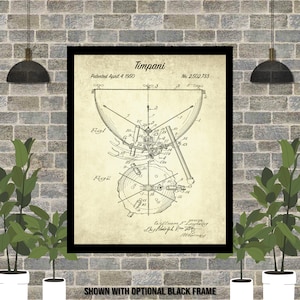This e-commerce style image showcases a framed black-and-white poster, set against a realistic backdrop of grey brickwork with plants symmetrically placed on either side. The poster, which appears to be an old-fashioned schematic drawing, has an optional black frame, as indicated by the small black text along the bottom. The drawing resembles a patent design, possibly for a timpani drum, featuring detailed illustrations labeled with numbers and the possible year "1890." Elements of the schematic include a large, bowl-shaped drum with a flat top, and various components detailed across the illustration. The product photo effectively demonstrates how this steampunk-inspired, timeless artwork might look when displayed on a wall.